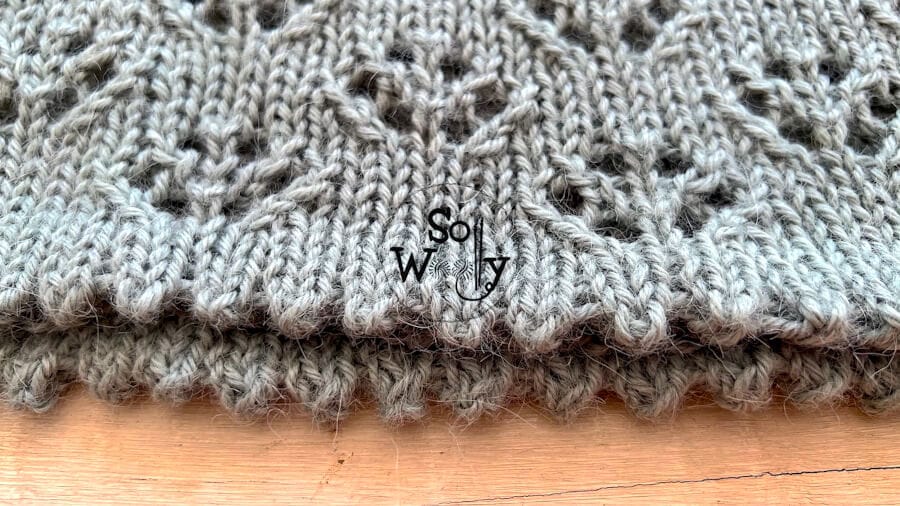This color photograph showcases a hand-knitted gray scarf made from various shades of yarn including light gray, white, and darker gray tones, resulting in a chunky texture. The scarf, intricately woven or knitted, features a scalloped edge at the bottom with a repeating floral or paw-print-like pattern running through its center. The edge of the scarf is folded over, revealing both the top and bottom layers, and highlighting the detailed yarn work. Centrally positioned in the image is a finely outlined emblem with the text "Sewoolee," where the 'O' is creatively depicted as a bundle of yarn, and the 'L' resembles a knitting needle, all encased within a circular border. This setup rests atop a light wooden floor, suggesting a cozy, warmly lit environment that possibly benefits from natural daylight streaming through a window.